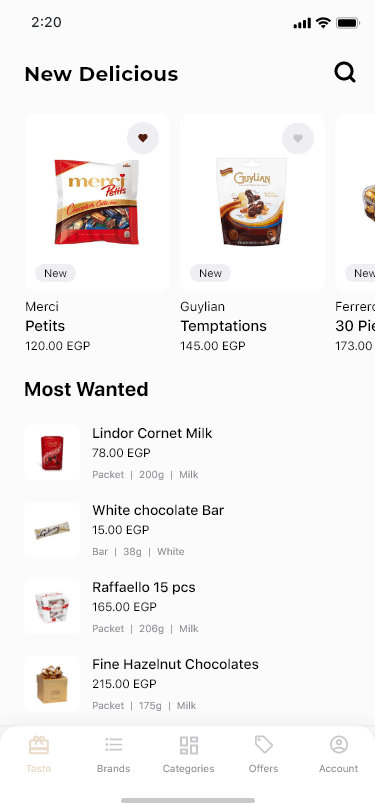The image features a screenshot of a shopping app interface. In the top-left corner, the time is displayed as 2:20. Adjacent to this on the right, there's a horizontal battery icon, colored black and nearly full.

Beneath the time, the text "New Delicious" is prominently displayed. To the right of this text, a search bar is located, facilitating user searches.

Below the search bar, three candy packages are showcased. The first is in red, white, and brown packaging, labeled with the word "New" and identified as "Merci Petites" priced at 120.00 EGP. Next to it on the right, there is another package of candy, this time appearing to be chocolate, branded as "GUYLIAN" and below that, the word "Temptations" along with the price of 145.00 EGP.

Further down, the label "Most Wanted" is visible, followed by a listing for a small red package of "Lindor Cornette Milk" priced at 78.00 EGP. Below this item, there is a "White Chocolate Bar" priced at 15.00 EGP.

Continuing downward, there is a package of 15 pieces of "Raffaello" priced at 165.00 EGP. Finally, at the bottom, a brown box containing "Fine Hazelnut Chocolates" is priced at 215.00 EGP.